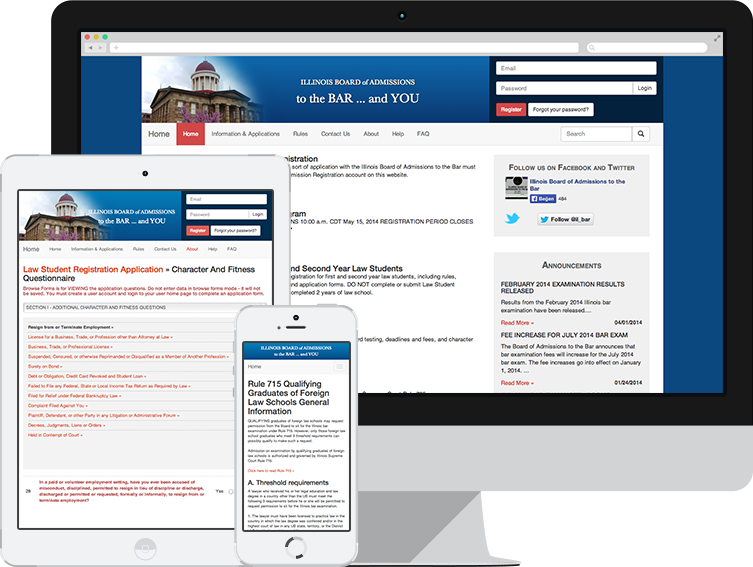The image showcases a range of Apple products displaying the Illinois Board of Admissions to the Bar website in various formats. Featured prominently, a large iMac with a widescreen monitor presents the full desktop version of the site, offering an expansive and detailed view typical for desktop users. Adjacent to it, an older model iPad is shown in portrait orientation, displaying the tablet version of the site, which strikes a balance by fitting more information than the mobile version while still being compact. Finally, an older iPhone model with noticeable bezels encloses the mobile version of the site, which condenses the content to fit the smaller screen. This setup highlights the responsive design of the website, ensuring usability across different devices, from desktops to tablets to smartphones. Each screen provides a glimpse into how users might interact with the site depending on their device, demonstrating a meticulous approach to accessibility and user experience.